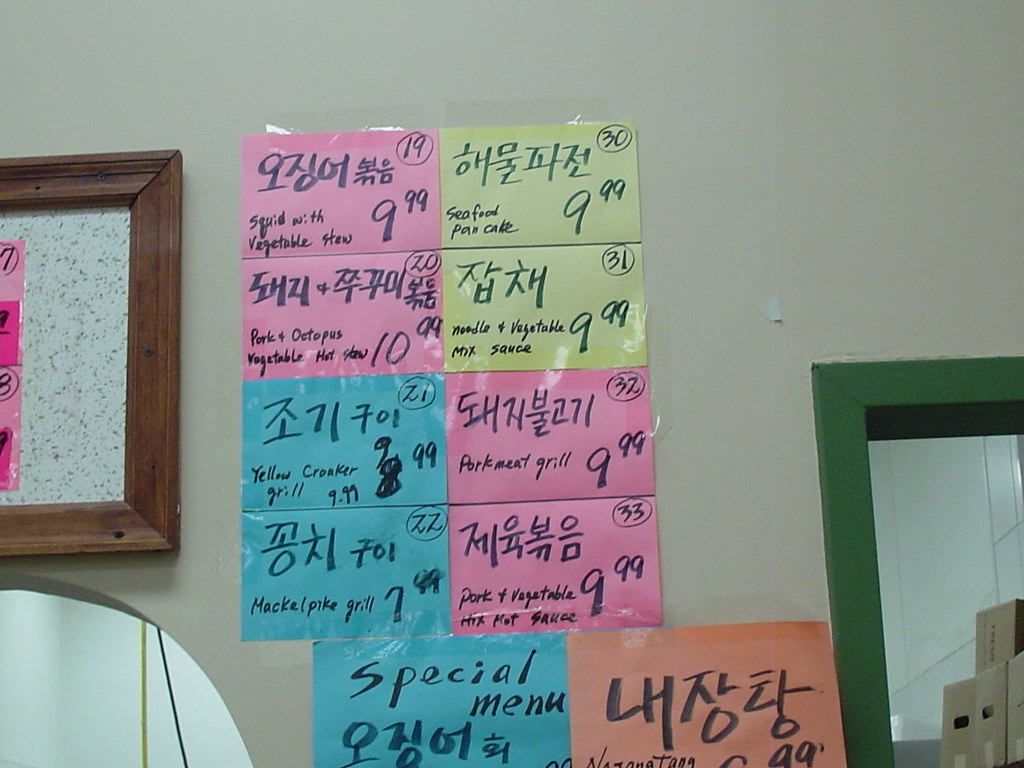The image showcases a basic yet vibrant restaurant menu, meticulously crafted from colorful notecards. These notecards, in shades of pink, yellow, blue, and a single orange, are neatly grouped together and mounted on an evidently aged white wall adorned with dark markings. The writing on the cards includes Japanese or Chinese characters with their English translations beneath each. The dishes listed include "Pork Meat Grill," "Pork Plus Vegetable," and "Pork and Octopus," with prices prominently displayed on the bottom right of each card, ranging between $7.99 and $10.99. Each card also features a circled number at the top right, likely indicating the order number, with figures such as 20, 21, 31, 32, 33, and 22. Adjacent to the menu display, a wooden picture frame is visible, its white interior flecked with brown. To the far right, a green door frame reveals the entrance to another room, adding depth to the quaint setting.